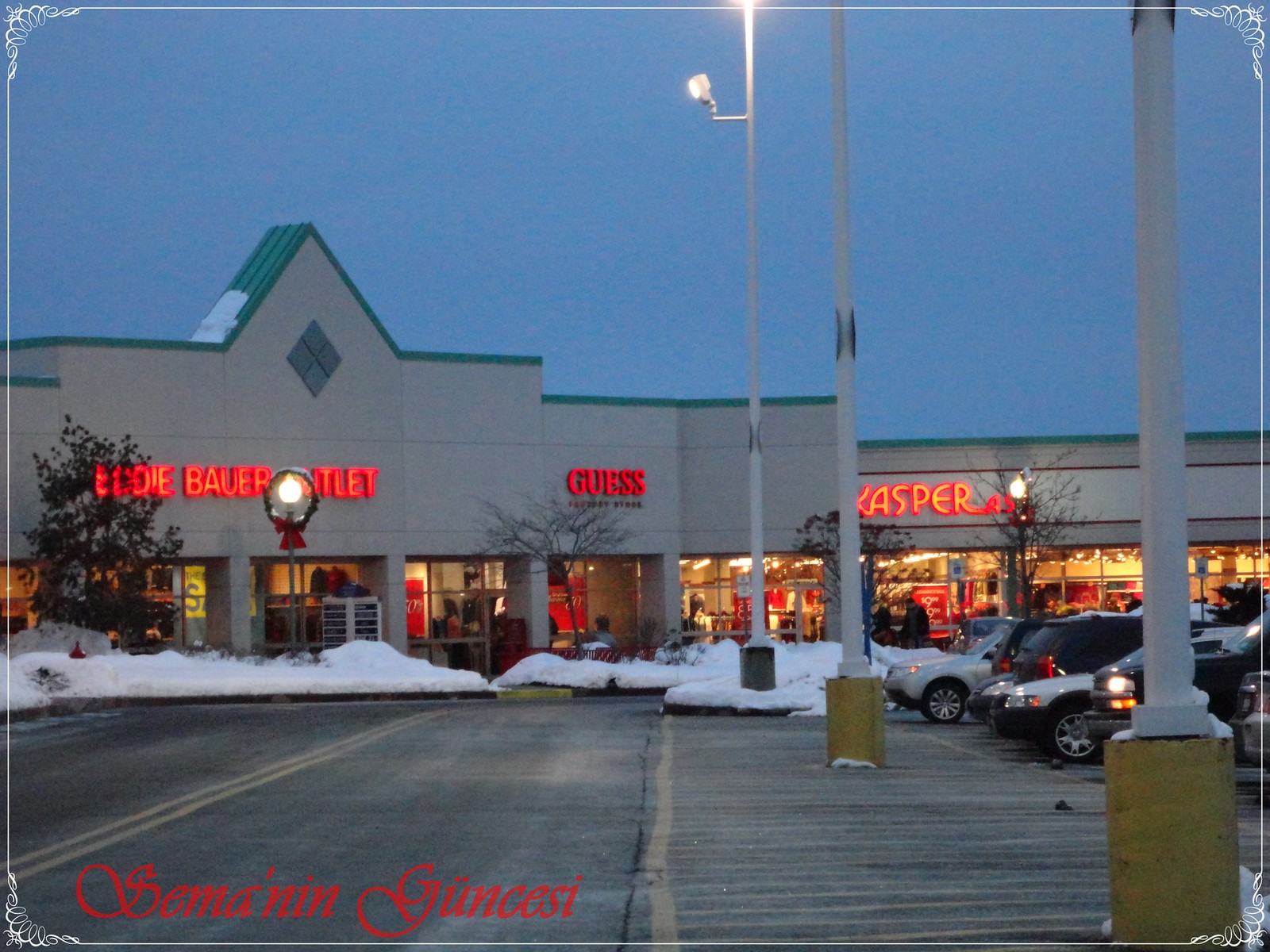This detailed photograph captures an outdoor strip mall in the early evening of winter. Evident from the snow piled up on the sides of the parking lot and sidewalks, which have been plowed, the strip mall itself features a white or off-white facade with a green top and a green checkered sign. The storefronts are illuminated with bright red signage, showcasing an Eddie Bauer Outlet on the left, a Guess store in the middle, and a Casper store on the right. Several cars are parked along the right side, near a road that leads into the parking lot and towards the stores. Streetlights on cement bases light the scene. A distinctive element of the image is a thin decorative frame and text in cursive, reading "Semanin Gunzesi," suggesting an exotic or foreign location.